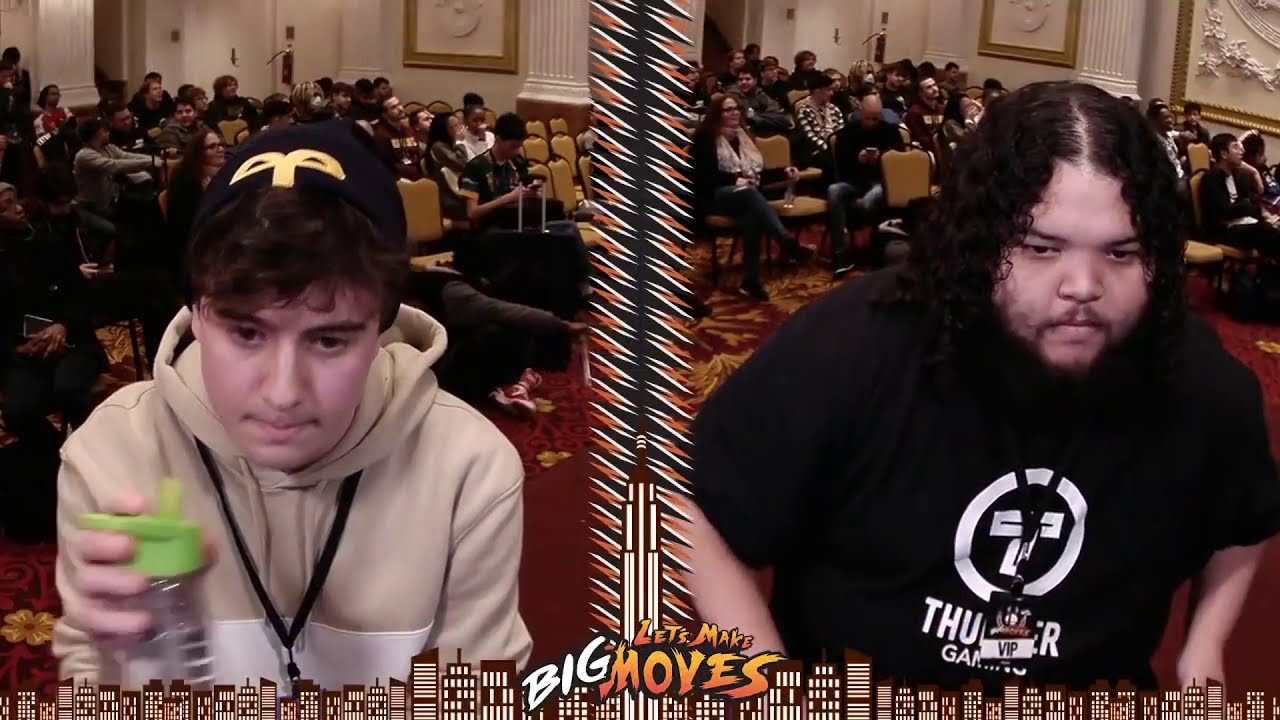In this photograph taken indoors, we observe two competitive gamers positioned in a split-screen layout. The image is three inches tall and six inches wide, divided by a vertical zigzag pattern down the center, featuring a thin narrow black diamond framed by red and white flames. The background consistently showcases a crowd of people seated in chairs, suggesting a lively convention-like setting. 

On the left side, a young Caucasian man with fluffy brown hair, a black beanie marked with a gold emblem, a tan hoodie with a white stripe, and holding a water bottle with a green lid is visible. Behind him, the seated audience can be seen, adding depth to the imagery.

On the right side is a man of probable Polynesian descent, with long, curly black hair parted in the center. He sports a short-sleeved black shirt adorned with white print, a lanyard with a VIP tag, a slight mustache, and a beard, reinforcing the competitive ambiance.

The bottom center of the photograph prominently displays the text "Let's make big moves" with "big" in white print and the rest in gold. Below this text, a cityscape with white-detailed windows can be seen, along with a towering structure defining the middle of the scene. The colors in the image include tan, green, white, black, yellow, and red, contributing to the vibrant competitiveness of the atmosphere, likely related to a video gaming event.